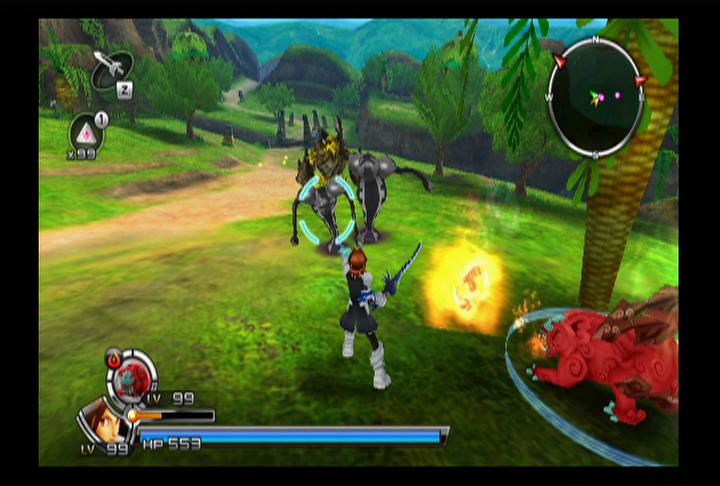In this vividly detailed image from a video game, a central character stands ready with a sword, embodying a fighter's stance. Approaching them are two unique characters: one resembles an insect with exaggerated eyes and ears, while the other appears to be a monstrous figure marked by a distinctive turquoise ring on its front, likely an in-game marker. A figure surrounded by yellow flames can be spotted nearby, adding to the dramatic scene. A palm tree bears an emblematic target, and within the marked inner circle of another marker stands a red, bull-like creature. The landscape includes a winding road, majestic mountains, and scattered trees. Various in-game elements and markers numbered "1" and "2" are sprinkled throughout the scene. At the bottom of the image, a user interface with a box displays bars and numbers, likely indicating player stats or game mechanics.